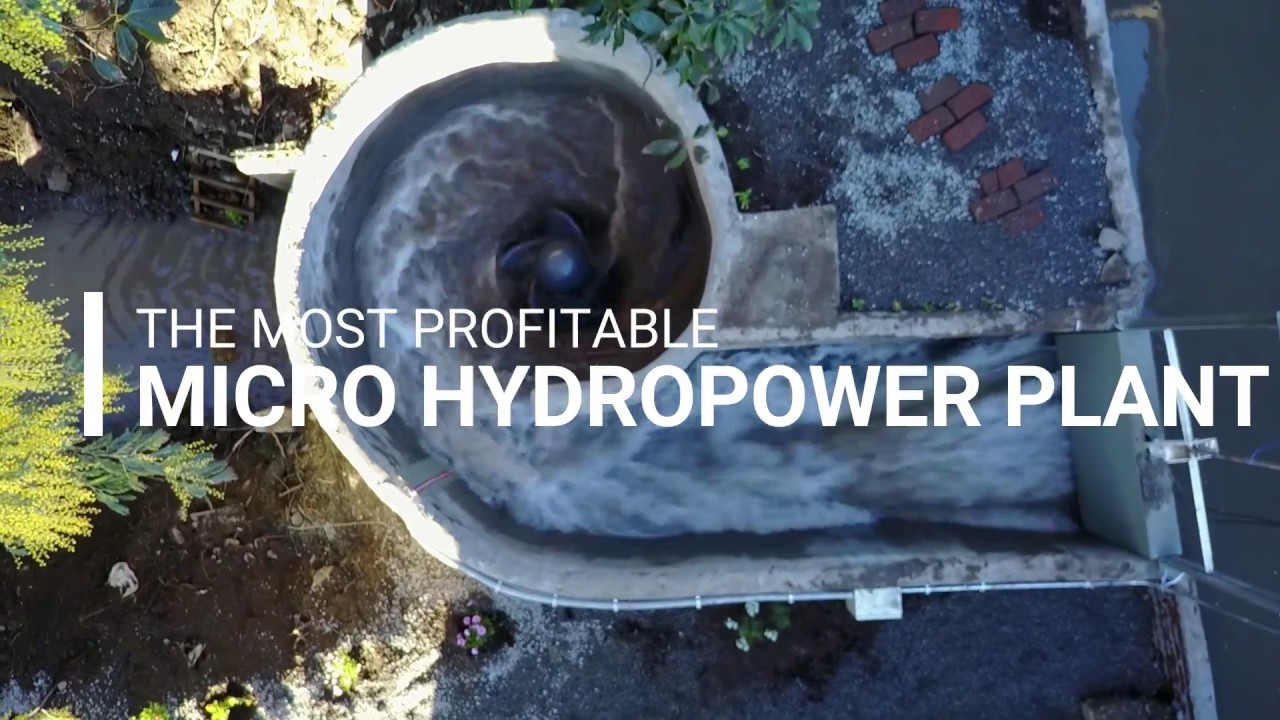The aerial photograph, likely taken from a drone during the daytime, prominently features the text "THE MOST PROFITABLE MICRO HYDROPOWER PLANT" in large white font across the image. At the center of the photo lies a circular whirlpool within a concrete bowl, which appears to be the hydropower plant. Water emerges from a partial wall, creating a circular motion before draining off to the right into a lower level, resembling a miniature river. Surrounding this focal point are various elements: piles of bricks, green shrubbery, and a small gate. The landscape includes scattered stones and trees, particularly visible on the left side of the image. The color palette is a mix of blue, gray, green, yellow, white, brick red, and dark gray, adding to the vivid and detailed composition of this outdoor setting.